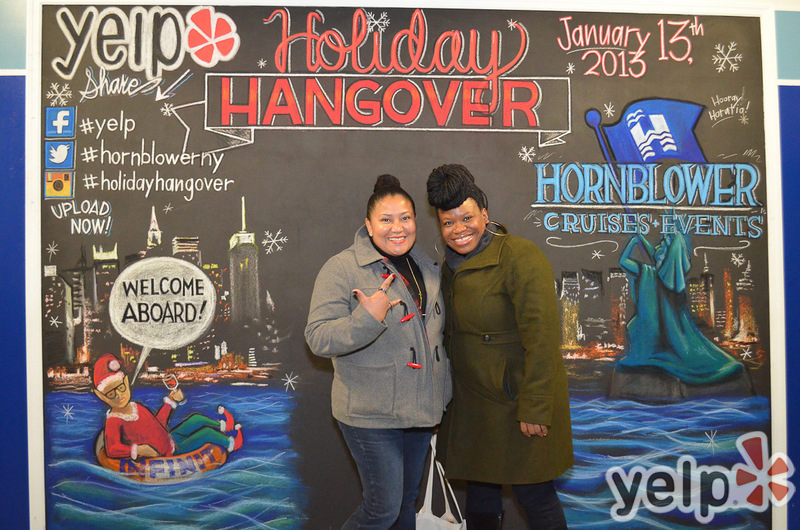The image captures two smiling black women posing in front of a vibrant and detailed mural that promotes Yelp and Hornblower Cruises Events. The woman on the left is wearing a grey jacket with red buttons and blue jeans, has black hair pulled into a ponytail, and is showing off her red nail polish. The woman to her right is dressed in a green coat with blue jeans. Both women are looking directly at the camera and appear cheerful. The mural behind them is adorned with colorful illustrations and multiple textual elements. At the top, the headline "Holiday Hangover" is prominently displayed in red lettering with a white outline, dated January 13, 2013. There are various social media icons and hashtags, including Yelp and Hornblower NY, scattered across the mural. In the lower right corner of the mural, an abstract drawing of the Statue of Liberty blowing a horn and holding a blue flag with a white "H" can be seen. Below it, the name "Hornblower Cruises Events" is written in light blue. The mural also features an elf wearing a Santa hat, red top, green pants, and red elf shoes, floating in an orange inner tube on water, raising a glass of wine with a speech bubble saying, "Welcome aboard!" Snowflakes and a cityscape form the background, contributing to the festive holiday theme.